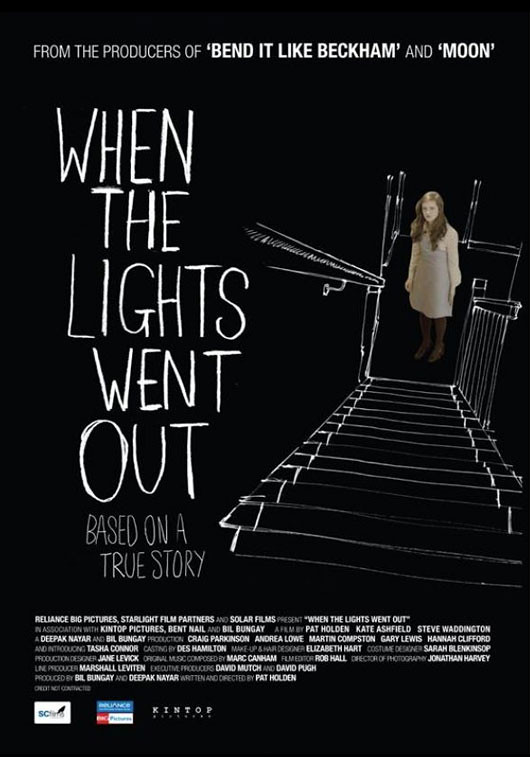The movie poster for "When the Lights Went Out" features a striking black background with white print. Across the top, it prominently states, "From the producers of Bend It Like Beckham and Moon." To the left side, written vertically in a handwritten-style font, is the film's title, "When the Lights Went Out," with the subtitle "Based on a True Story" just beneath it in a lighter white font. In the upper right portion of the poster, an illustrated image depicts a narrow staircase in a house, viewed from the top down, complete with a railing and banister. At the bottom of this staircase stands a girl, depicted in full color, contrasting against the monochrome setting. She has long light brown or auburn hair cascading over her shoulders. Her outfit is a knee-length, long-sleeved beige dress, paired with brown stockings and brown shoes. The girl is gazing upward toward the top of the staircase. Below the illustration, at the poster’s bottom, there is additional information in small text about the film’s cast and crew, accompanied by logos of the production and distribution companies.